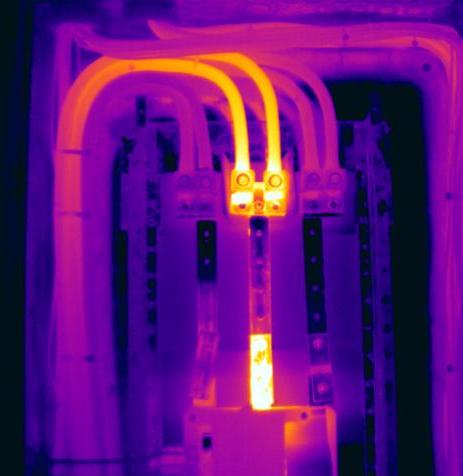In a photograph that appears intentionally blurred, an intricate, industrial-looking electrical contraption is adorned with vibrant neon lights in shades of yellow, purple, pink, and orange. The background is pitch black, making the neon colors stand out starkly. The lights, shaped like thick piping or tubing, form a rigid, geometric square. Despite its seemingly abstract nature, the scene hints at an industrial setting where mechanical components seem to interact. The overall composition suggests an artistic modification, likely altering the natural colors to emphasize an aesthetic or thematic element. No identifying information is present to clarify the contraption's purpose, location, or the nature of the image—whether it is a photograph, a digital drawing, or possibly a still from a film.